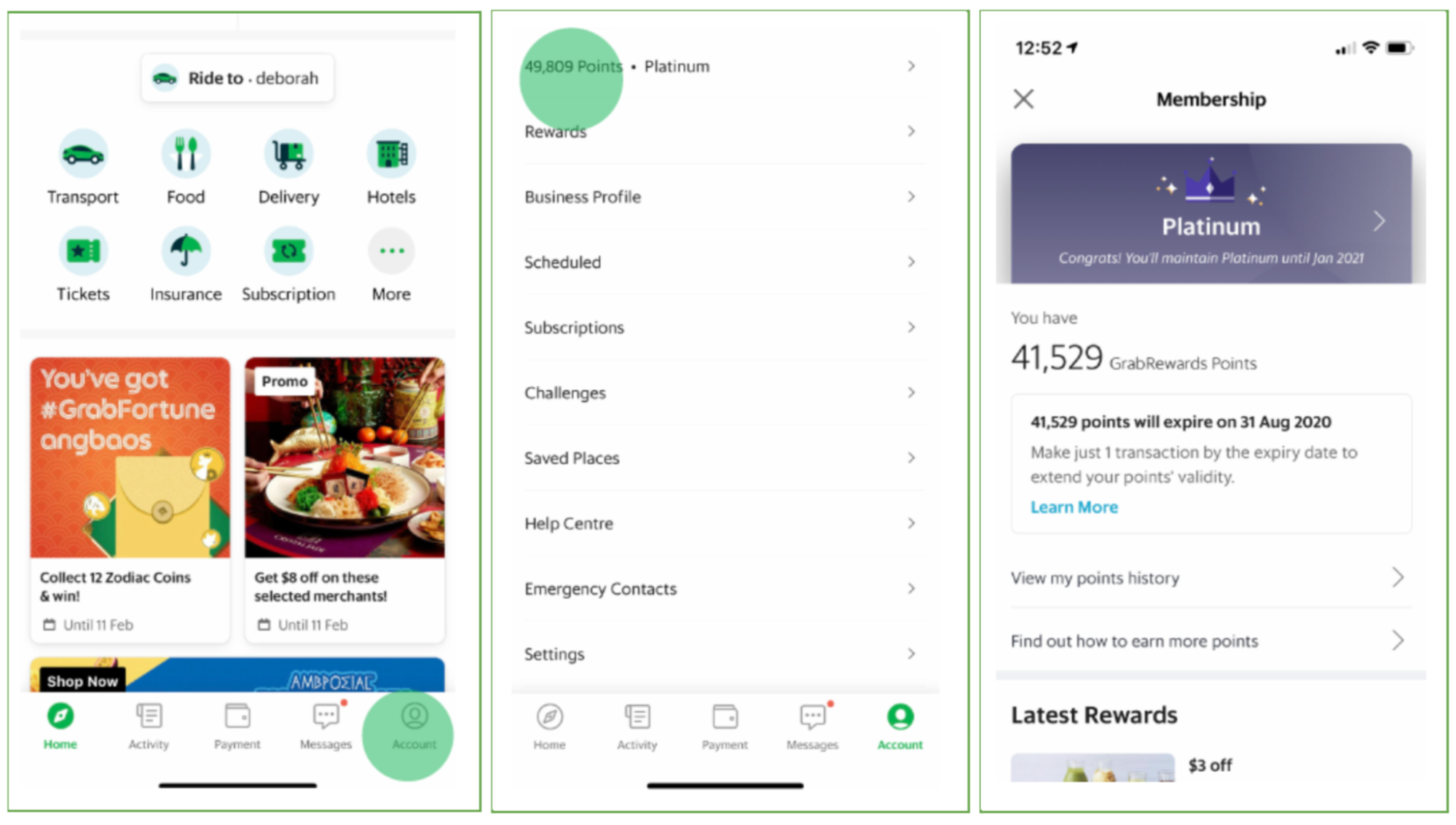This image depicts a detailed layout of a website interface, likely associated with a mobile app. The interface appears to be split into three sections or screenshots, each showcasing different features and information.

### Screenshot 1: Ride and Promotional Offers
**Header:**
- A circular profile picture in the center displaying a car.
- "Ride to" with the name "Deborah" beneath it.

**Icons:**
- A series of eight icons below: 
  - Car (Transport)
  - Fork and Spoon (Food)
  - Hand Truck (Delivery)
  - Large Building (Hotels)
  - Ticket (Tickets)
  - Umbrella (Insurance)
  - Piece of Paper or Subscription (unclear icon)
  - Three dots in a row (More)

**Promotional Section:**
- Two images below the icons: one is a computer-generated advertisement, and the other is a photo.
  - **Ad Description:** 
    - Text: "You've got #GrabFortune ANGBaOS"
    - Background: Orange with a green square and an envelope, accompanied by small animal-like figures in circles.
  - **Photo Description:**
    - A restaurant scene with three people using chopsticks, suggesting an Asian eatery.
    - Text: "Get $8 off on these selected merchants, until 11 February."

**Additional Information:**
- **Promotional Details:**
  - "Collect 12 Zodiac coins and win," with a small symbol indicating the offer validity until 11 February.

**Navigation Bar:**
- Located at the bottom, with icons for Home (selected), Activity, Assignment, Messages, and Account.

### Screenshot 2: Rewards and Settings
**Top Section:**
- Display shows "49,809 points" with a green circle indicating "Platinum."

**List Items:**
- An extensive list including:
  - Rewards
  - Business Profile
  - Scheduled
  - Subscriptions
  - Challenges
  - Saved Places
  - Help Center
  - Emergency Contacts
  - Settings

**Navigation Bar:**
- Identical to the first screenshot.

### Screenshot 3: Membership and Points
**Top Bar:**
- Time: "12:52"
- Signal strength: 2 out of 4 bars
- Wi-Fi symbol
- Battery level: Approximately 90%

**Membership Information:**
- Title: "Membership"
- Icon: Credit card with a crown labeled "Platinum."
- Text: "Congratulations, you'll maintain platinum until January 2021. You have 41,529 Grab Rewards points. 41,529 points will expire on 31 August 2020. Make just one transaction by the expiry date to extend your points' validity."

**Links and Rewards:**
- Clickable links:
  - "Learn more"
  - "View my points history"
  - "Find out how to earn more points"
  - "Latest rewards"

Overall, this image represents a rich, multifaceted user interface displaying ride information, various services and promotions, user rewards, membership status, and system navigation tools.